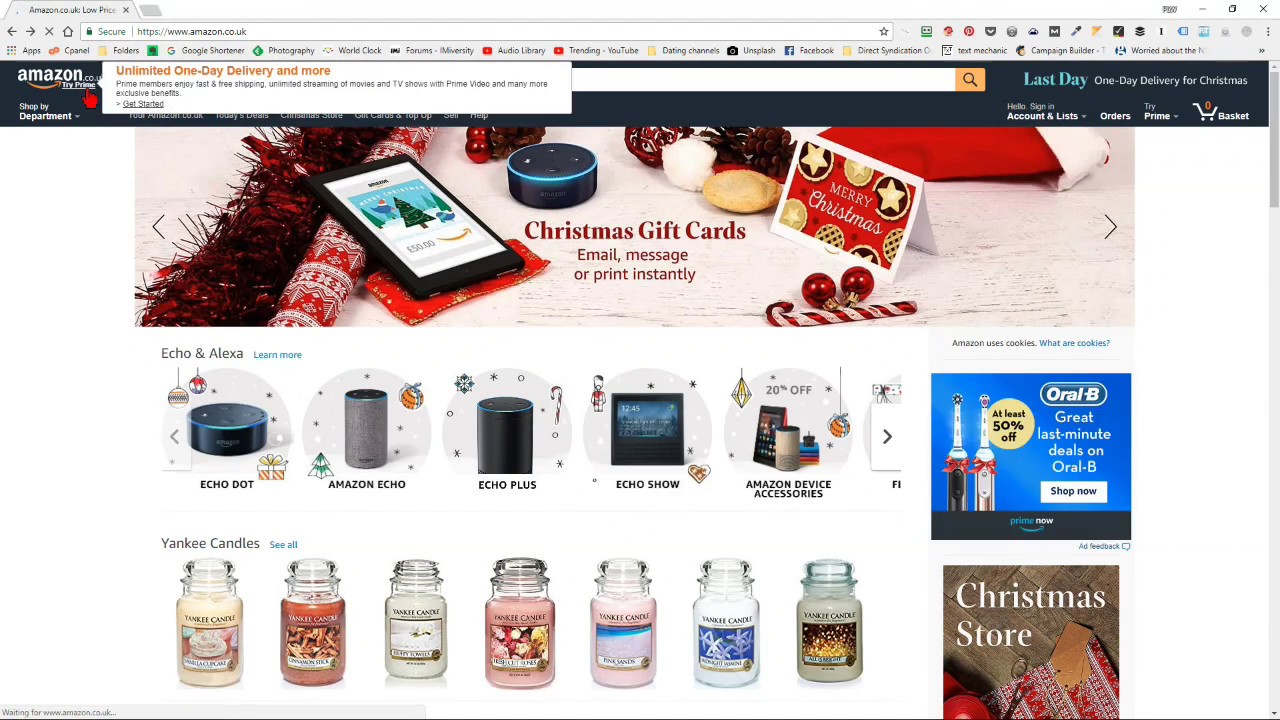**Caption:**

An Amazon webpage offering last-minute Christmas deals is displayed against a white background. The center of the screen features a shopping cart icon with an orange "0" inside, indicating an empty cart. Multiple navigational tabs are visible, including a prominent "Try Prime" button in white and gray, and an "Orders" tab also in white. The "Hello, Sign In" greeting is shown in gray. 

At the top, a banner announces "Unlimited One-Day Delivery and More" in orange. Below this, there are Christmas-themed gift cards with a "Merry Christmas" message, available for email, message, or instant print. 

The page showcases various gift ideas, including a candy cane-wrapped iPad, a stocking filled with cookies, and Amazon devices like the Echo Dot, Echo, Echo Plus, and Echo Show, with a prompt to "Learn More" in blue. A section promoting Amazon device accessories offers a 20% discount. Additionally, discounts on Yankee candles, featuring seven different scents, are highlighted.